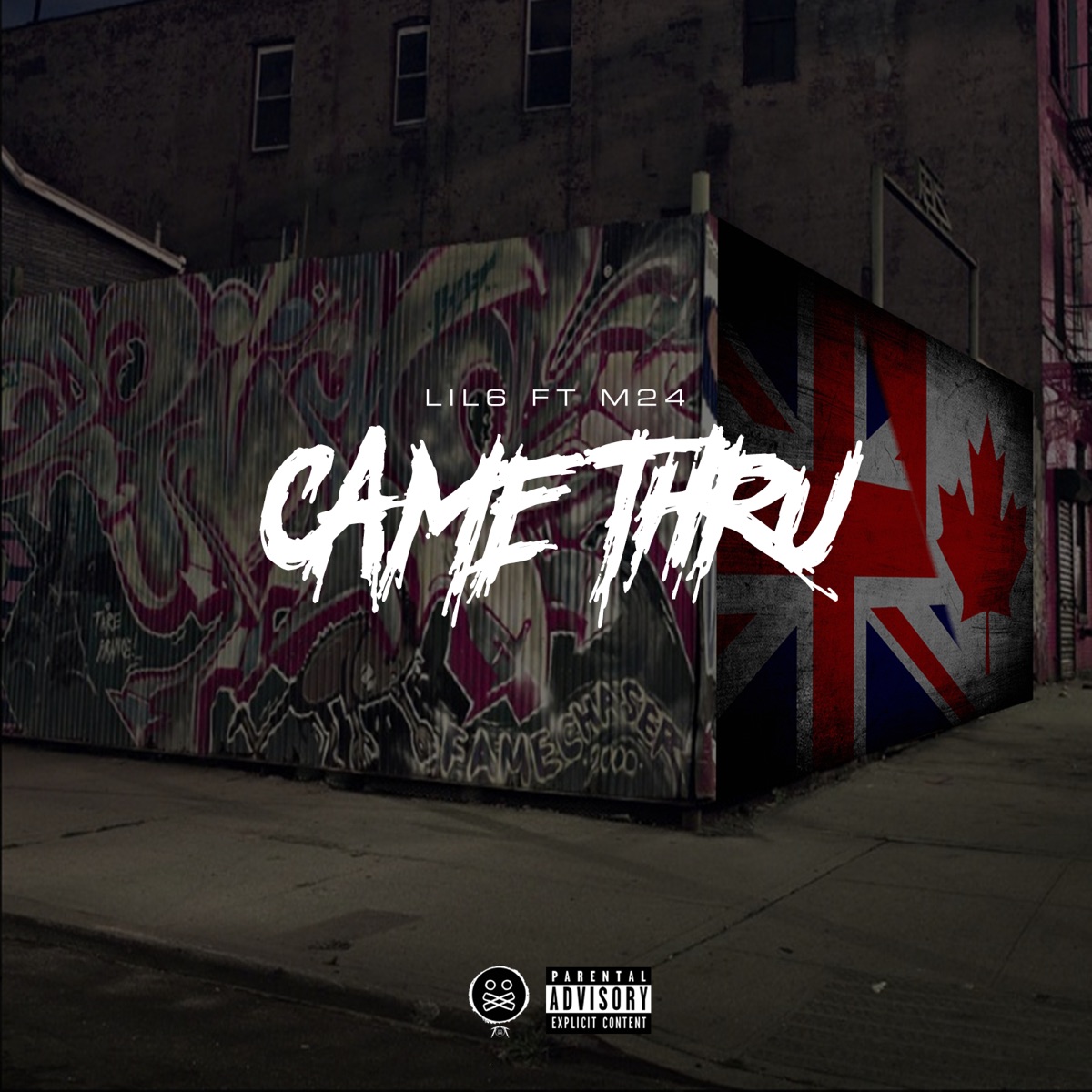The image appears to be a stylized CD cover, presenting a gritty and urban aesthetic. It features a detailed depiction of a street corner, framed by two adjoining walls forming a slight vertical rectangle. The left wall is heavily adorned with graffiti, predominantly in purple and white, with various designs and the phrase "Fame Chaser" inscribed at the bottom right. The right wall displays partial illustrations of the British and Canadian flags— the British flag's red cross with white lines and the Canadian flag’s red maple leaf on a white background. 

Dominating the center of the image is bold, aggressively brush-stroked white text that reads "Game Through," styled to appear as though painted with thick, violent strokes, some splashing beyond their intended lines. Above this text, the tag "LIL6FTM24" is positioned, while at the bottom center, there's an emblem adjacent to a black rectangular sticker indicating "Parental Advisory: Explicit Content." The colors in the image are mainly dark shades of black and gray with splashes of white, red, and blue, contributing to the overall edgy and provocative atmosphere.